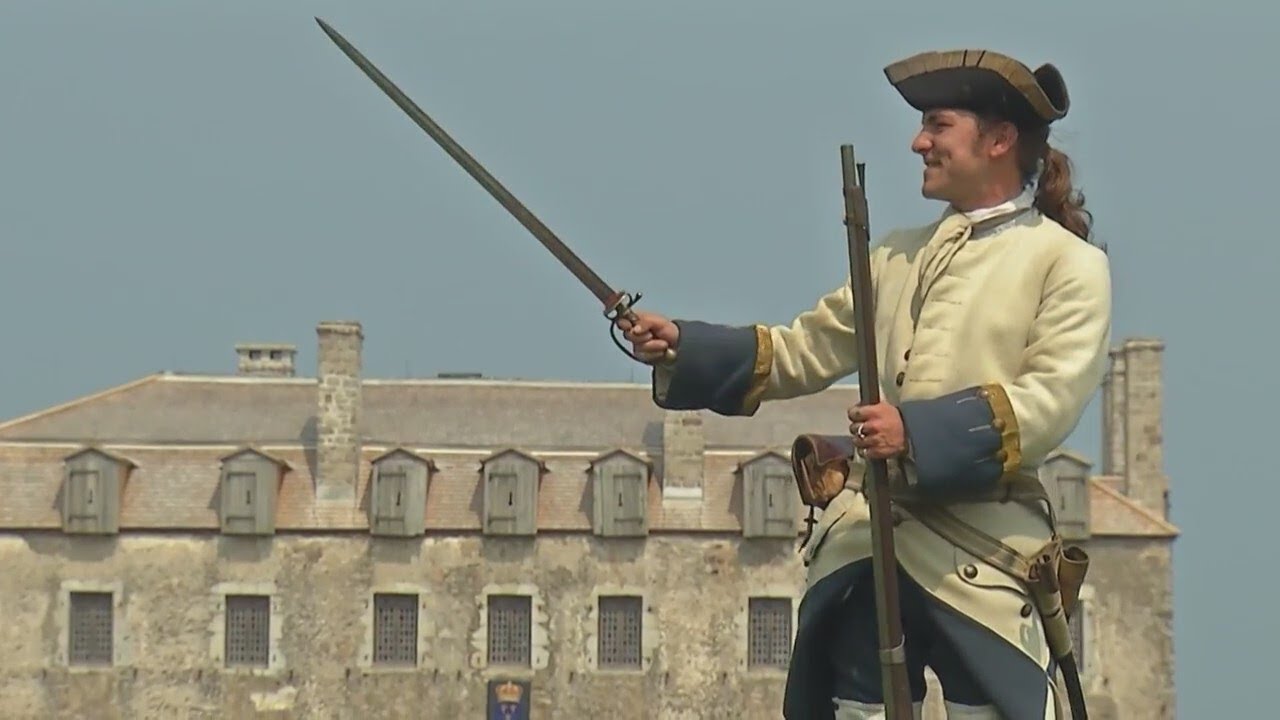In this outdoor, daytime color photograph, an individual dressed as a Revolutionary War soldier stands in front of an old cement and stone building with a dull, overcast sky overhead. Positioned in the lower right-hand corner of the horizontal frame and facing left, the man is captured in profile with detailed emphasis on his colonial attire. His costume features a cream-colored shirt with large, flowy blue and gold sleeves, and matching blue pants, topped off with a traditional blue and gold Revolutionary War hat. His long, light brown hair is tied back in a ponytail, and he is approximately in his thirties, with a strong chin and nose visible in his profile. 

In his right hand, which is extended to chest level, he holds a meter-long sword poised as if ready for action. His left hand grips a musket, the butt of which rests on the ground, making it unusable in his current stance. Attached to his hips are various pouches, complementing his historically inspired outfit. The backdrop reveals a classical style building with multiple windows, including distinctive house-shaped and rectangular ones, and a visible chimney near the man's shoulder, adding to the authentic, vintage ambiance of the scene.